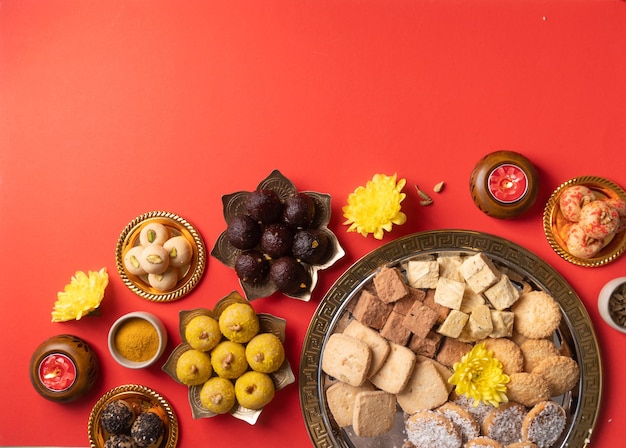This image depicts an ornate dessert table laden with an assortment of pastries and fruits, set against a vivid red background. In the bottom left corner, there is a small, round gold plate holding three treats. Above it, a yellow flower sits beside a patch of yellow powder. Below the powder, a gold flower-shaped dish contains seven yellow treats. Adjacent to this, another similar dish holds seven purple fruits. Just off to the left of these, a small round gold plate is adorned with five distinct treats. Moving to the bottom right, the setup features a gold plate with three more treats, a nearby flower, a candle, a bowl of nuts, and a larger plate brimming with an assortment of cookies, pastries, and a little yellow flower. The arrangement, featuring Oriental design elements such as the intricate flower dishes and the decorative candles, evokes a sense of a carefully curated Oriental dessert display.